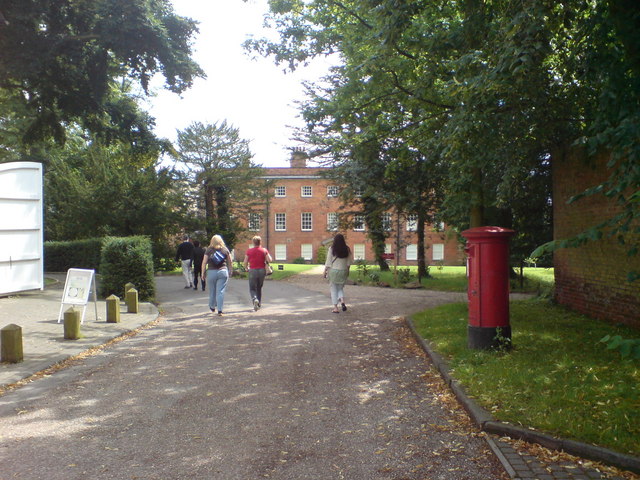The photograph captures a college campus scene with a group of five casually dressed individuals walking away from the camera towards a large, three-story brick building characterized by its numerous white-framed windows. The path they are walking on appears to be either gravel or rocky pavement and is shaded by numerous trees, creating a tranquil atmosphere. On the right side of the street, there's a small grassy area partially shaded by trees, where a prominent red fire hydrant stands near a brick wall covered in ivy. This grassy patch is also home to a series of cement stubs or small pillars, possibly serving as seating areas. To the left side of the path, the street is bordered by bushes, enhancing the lush, green surroundings. The individuals, consisting of three women and two men, are dressed in light, casual attire, indicating a warm day. The women are seen holding handbags or wearing backpacks, and their outfits range from dark shirts to blue jeans, black pants, and a skirt with leggings. The scene exudes a peaceful, scholarly environment reflective of a well-tended college campus.